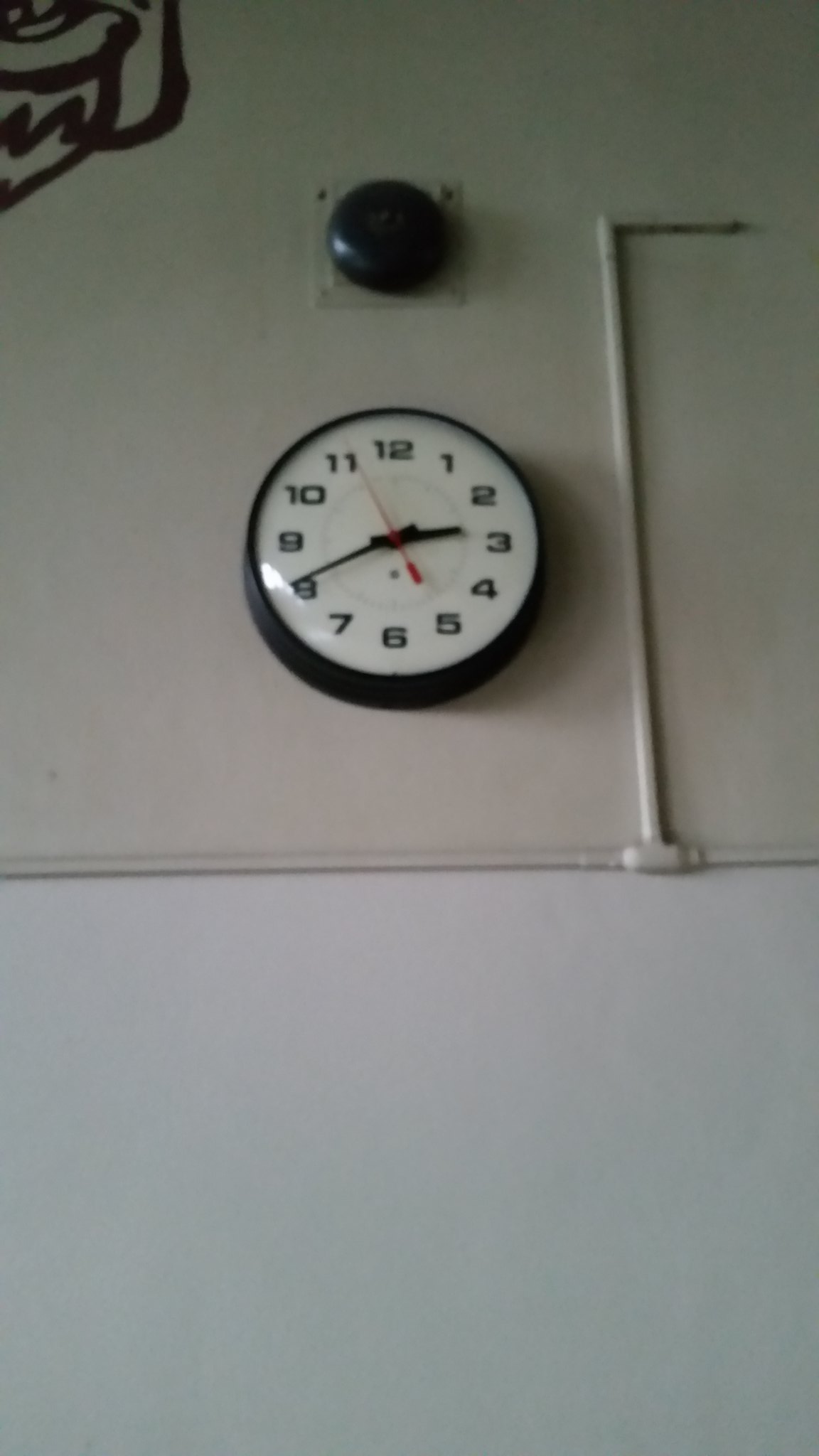This photograph captures a round clock mounted on a pristine white wall. The clock features a white face with one red hand and two black hands indicating the time against prominent black numbers. A glass cover on the clock face reflects light, adding a subtle gleam to the image. To the right of the clock, there's a narrow white vertical strip that slightly veers off to the side. Above the clock, a gray-toned bell is visible, adding an element of vintage charm. The wall above and to the right of the bell reveals a partial view of a brown-hued object. Additionally, the clock casts a distinct, circular shadow on the white wall, enhancing the overall depth and dimension of the photograph.